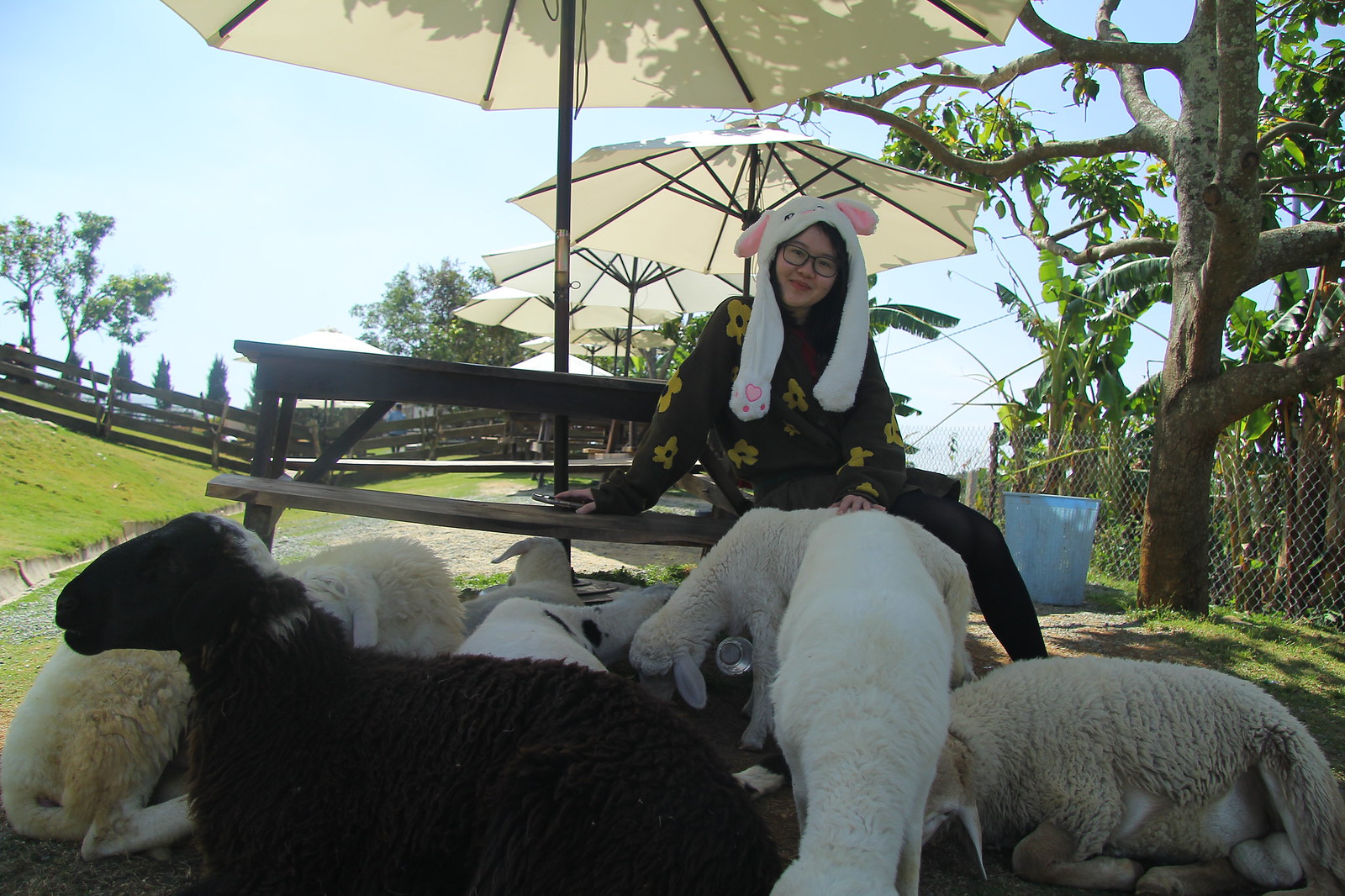In this outdoor scene on a sunny day with a bright blue sky, a woman is sitting on a park bench with a built-in white umbrella providing shade. She is wearing glasses and a distinctive white furry hat with pink ears and black dots, resembling a sheep, along with a black shirt adorned with yellow flowers. She is located in a lush, grassy area with multiple similar benches and umbrellas behind her. Nearby, grazing in the grass, are several lambs—most of them white, with one black, and a couple that might be beige. To the left, there's a grassy hill with a wooden walkway and wooden banisters, and a ditch in front of it. A road with a fenced area full of tropical-looking trees runs adjacent to the scene, while a tree trunk, a blue waste can, and additional trees can be seen in the background, creating a serene and picturesque setting.